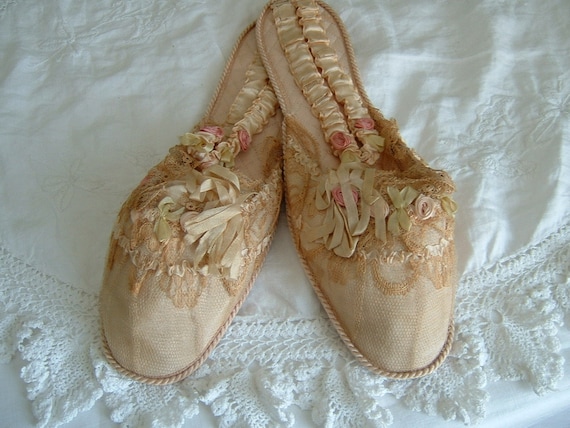The image showcases a detailed, top-down photograph of a pair of well-used, tan-colored ballerina shoes, which might also be perceived as slippers. Each shoe, positioned in the center of the frame with the right one's heel overlapping the left's, is adorned with delicate fabric flowers—approximately five pink, rose-like decorations on each. The shoes exhibit a soft, beige hue, possibly slightly darkened to an egg-white shade, and are elegantly narrow with curved toes. The interior of the shoes features ribbony, cushioned material for added comfort. The backdrop consists of a pristine, white tablecloth with frilly, lacy borders, contributing to the image's overall clean and well-lit appearance.